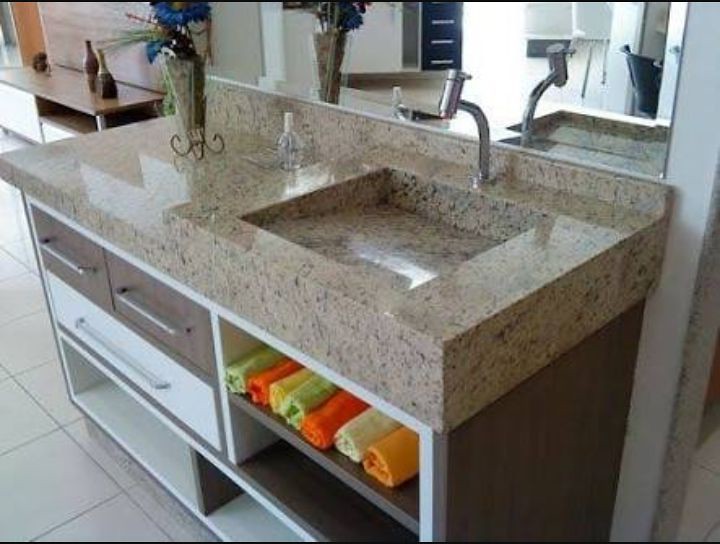The image depicts a section of a bathroom, the setting of which—whether in a business or a home—remains indeterminate. The centerpiece is a large mirror that dominates the upper portion of the image. Below the mirror sits an elegant light tan countertop, likely made of granite or stone, featuring dark speckles and swirls. The faucet boasts a long neck with a unique single-handle design at the top for twisting.

On the countertop, a clear vase with foliage stands on a pedestal, accompanied by a clear bottle with a spray top. Below the countertop are two brown drawers and several shelves, some brown and some white-trimmed. A rolled-up towel is visible on one of the shelves.

To the left of the countertop appears to be a vanity area, discernible by the presence of decanters or vases, and possibly a white chair. The mirror reflects parts of the bathroom's background, including drawers, a portion of the wall, and another chair, though the details are somewhat ambiguous.